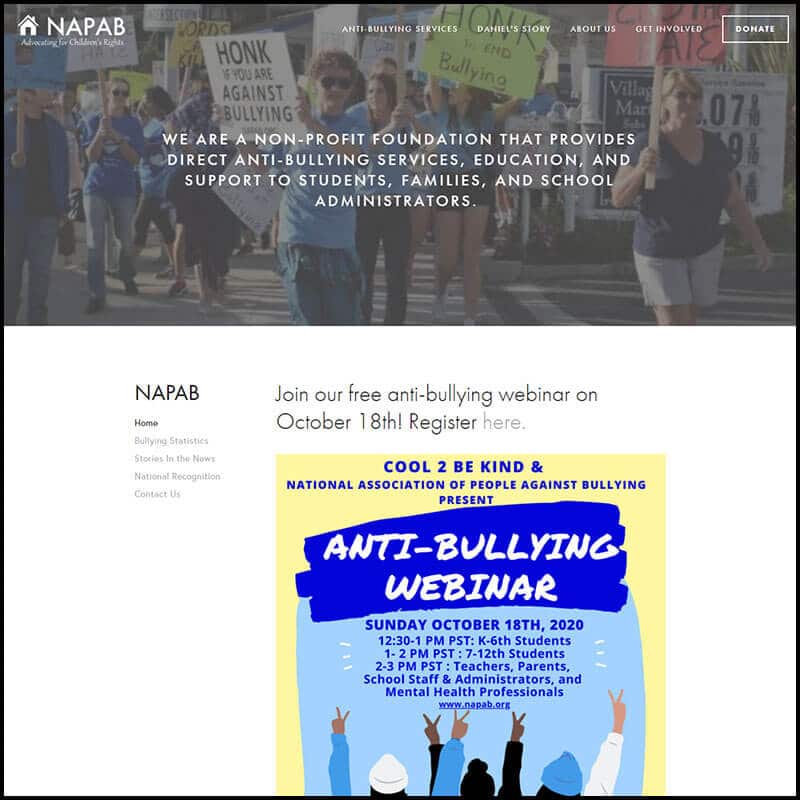This image depicts the homepage of the NAPAB (National Association of People Against Bullying) website. In the top left corner, "NAPAB" is prominently displayed next to a house icon, indicating the home page. Underneath, a slogan in white text states, "Advocating for Children's Rights." The upper section of the page features a background image showing people participating in a protest, holding signs with messages such as "Honk if you are against bullying" and "Honk to end bullying," the latter written on a yellow sign.

Below the background image, the main content of the website appears against a white background. In black text, an announcement invites visitors to "Join our free anti-bullying webinar on October 18th. Register here." Beside this, the acronym "NAPAB" is displayed in bold, black capital letters. Below this header, there are several navigational links, including "Home," "Bullying Statistics," "Stories in the News," "National Recognition," and "Contact Us."

At the center of the webpage is a flyer promoting the organization’s anti-bullying webinar. It reads, "Cool to be Kind and National Association of People Against Bullying present an anti-bullying webinar," styled in blue and white text against a background that blends blue and yellow hues.